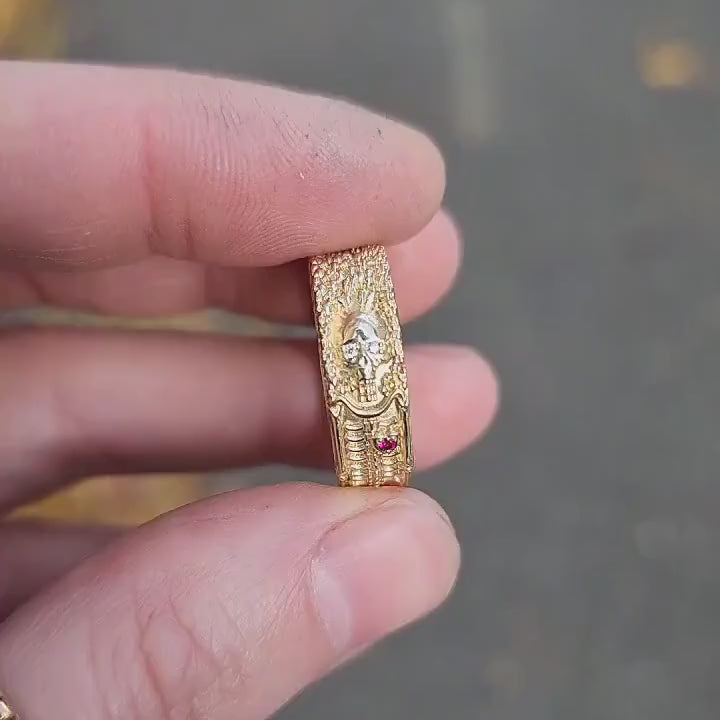In this realistic and square-shaped photograph, the focal point is a detailed left hand of an adult with white skin, emerging from the left side of the image. The background is a blurry, gray surface that could be a floor or ground, with slight touches of yellow. The hand, positioned in the foreground and in sharp focus, is holding a small, rectangular gold charm or ring between the thumb and index finger. The charm is intricately designed, featuring a protruding white skull at its center. Below the skull, there's an area with a different texture and a hint of red, possibly a ruby or similar jewel embedded in it. The ring, while nicely crafted, doesn't exude luxury. The setting suggests a simplistic yet intriguing scene with no accompanying text.